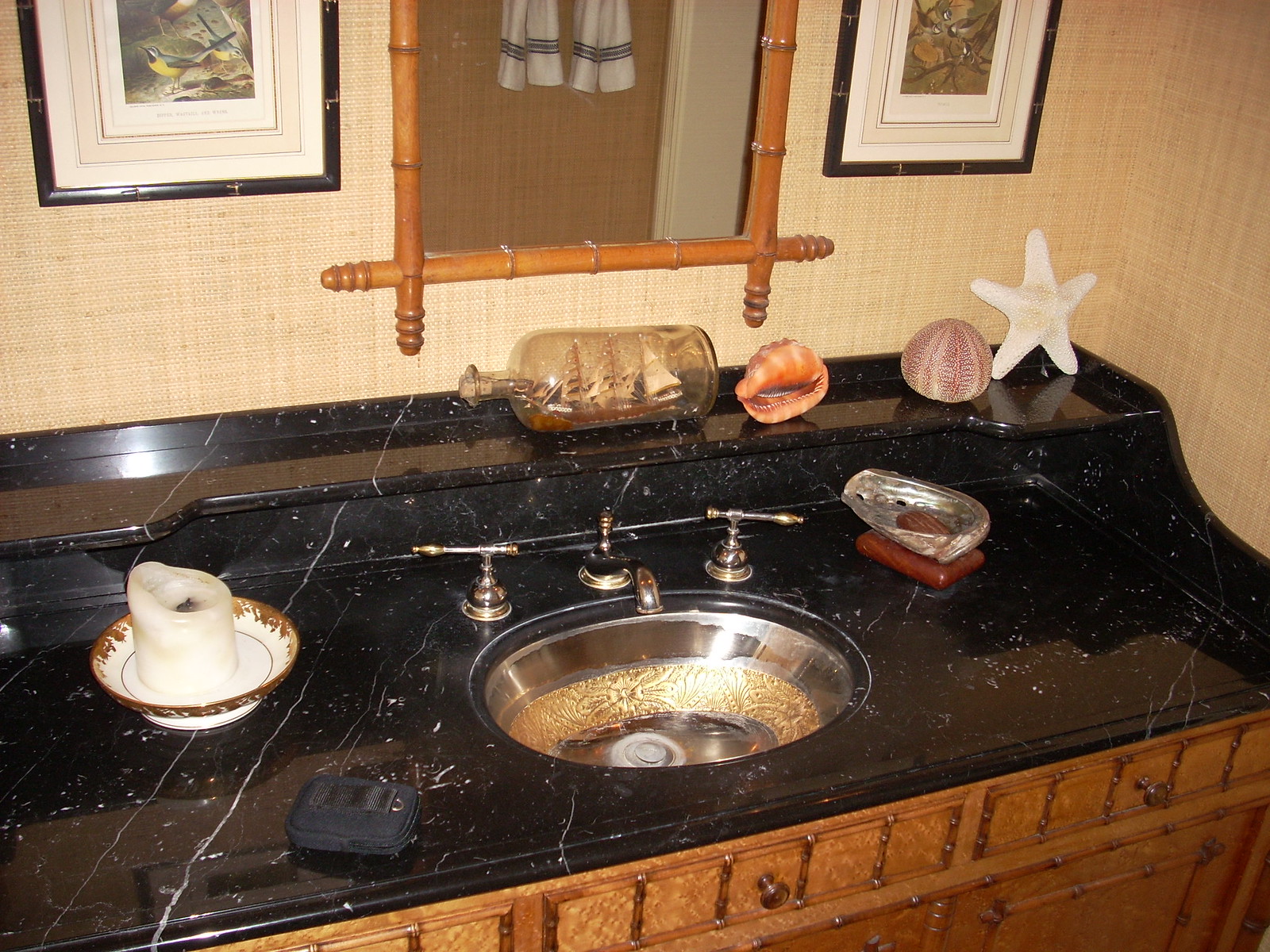This photograph captures a section of a tastefully decorated bathroom. The walls are adorned with a light tan wallpaper featuring a subtle grid pattern of vertical and horizontal lines. Flanking the bottom half of an elegant mirror, which has a distinctive bamboo frame, are two framed pictures. The left picture, encased in a black frame, depicts a vibrant yellow and blue bird. The right picture, also black-framed, showcases an orange flower with brown stems.

Reflected in the mirror are a few towels neatly hanging, white in color with blue stripes along the bottom. The vanity below the mirror features a sleek black marble countertop. Atop the counter sits a whimsical ship in a bottle, accompanied by an array of seashells and a starfish, adding a nautical touch. The sink is stainless steel with an ornate gold band around the middle, complemented by a brown cabinet below that features bamboo detailing.

Adding to the ambiance, a white candle housed in a white and gold dish, has been partially burned, indicating use. To the right of this, a glass soap dish shaped like a shell rests on a wooden base, adding elegance and a cohesive beach-inspired theme to the overall decor.